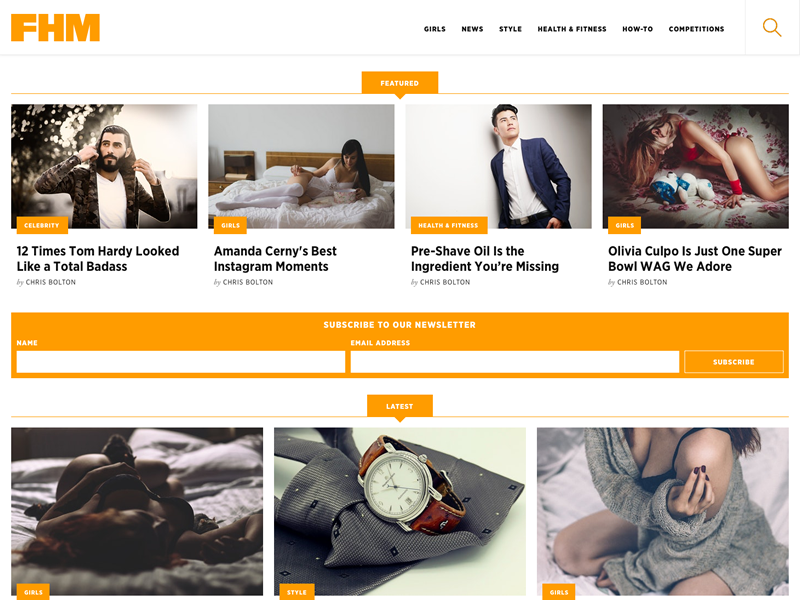This is a detailed description of the homepage for FHM. In the top left corner, you will find the FHM logo displayed in an orange hue. Moving across the page from the middle to the right edge, various categories are listed: Girls, News, Style, Health, Fitness, How-To, and Competitions. Adjacent to these categories, there is a magnifying glass icon indicating a search function.

Beneath these categories, featured articles are presented, including titles such as "12 Times Tom Hardy Looked Like a Total Badass," "Amanda Cerny's Best Instagram Moments," "Pre-Shave Oil Is the Ingredient You're Missing," and "Olivia Culpo: Just One Super Bowl WAG We Adore," the latter accompanied by an appealing image.

Below the featured articles, there is a prominent orange box, matching the logo's color, containing two fields for entering a name and email address to subscribe to the newsletter. A submit button is positioned next to these fields.

Further down the page, there are three pictures: the first depicts a woman lying on a bed, although the dim lighting makes it unclear whether she is asleep; the second shows a neatly arranged tie with a watch laid upon it; and the third picture features a woman kneeling on a bed, her face not visible, but highlighting her cleavage with a partially off-shoulder shirt, displaying a bit of her thighs.